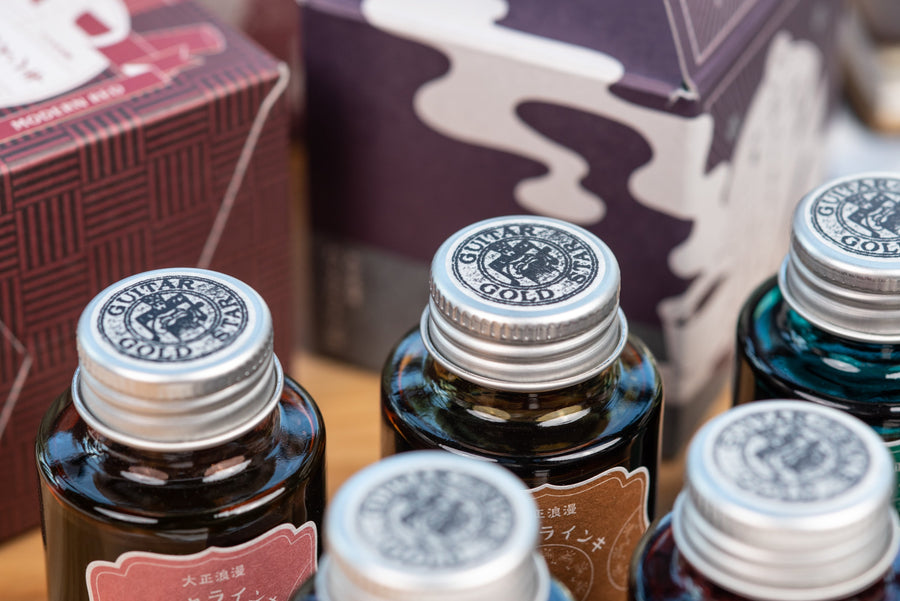The image displays an up-close shot of five small amber-colored glass bottles with aluminum lids, each labeled "Guitar Gold Star" with an image of a person playing a guitar. These bottles are neatly aligned, with three positioned in the back row and two slightly blurred in the front. The background is slightly out of focus, featuring a couple of tissue boxes—one with a red and black design and the other sporting a purple and white splotchy pattern. To the left, there's a brown box with white squiggly designs. The labels on the front of the bottles are written in a language that appears to be either Chinese or Japanese. The photograph seems to be taken at a market sale, capturing these items intended for guitar maintenance, possibly guitar oil, emphasizing their availability and distinct packaging.